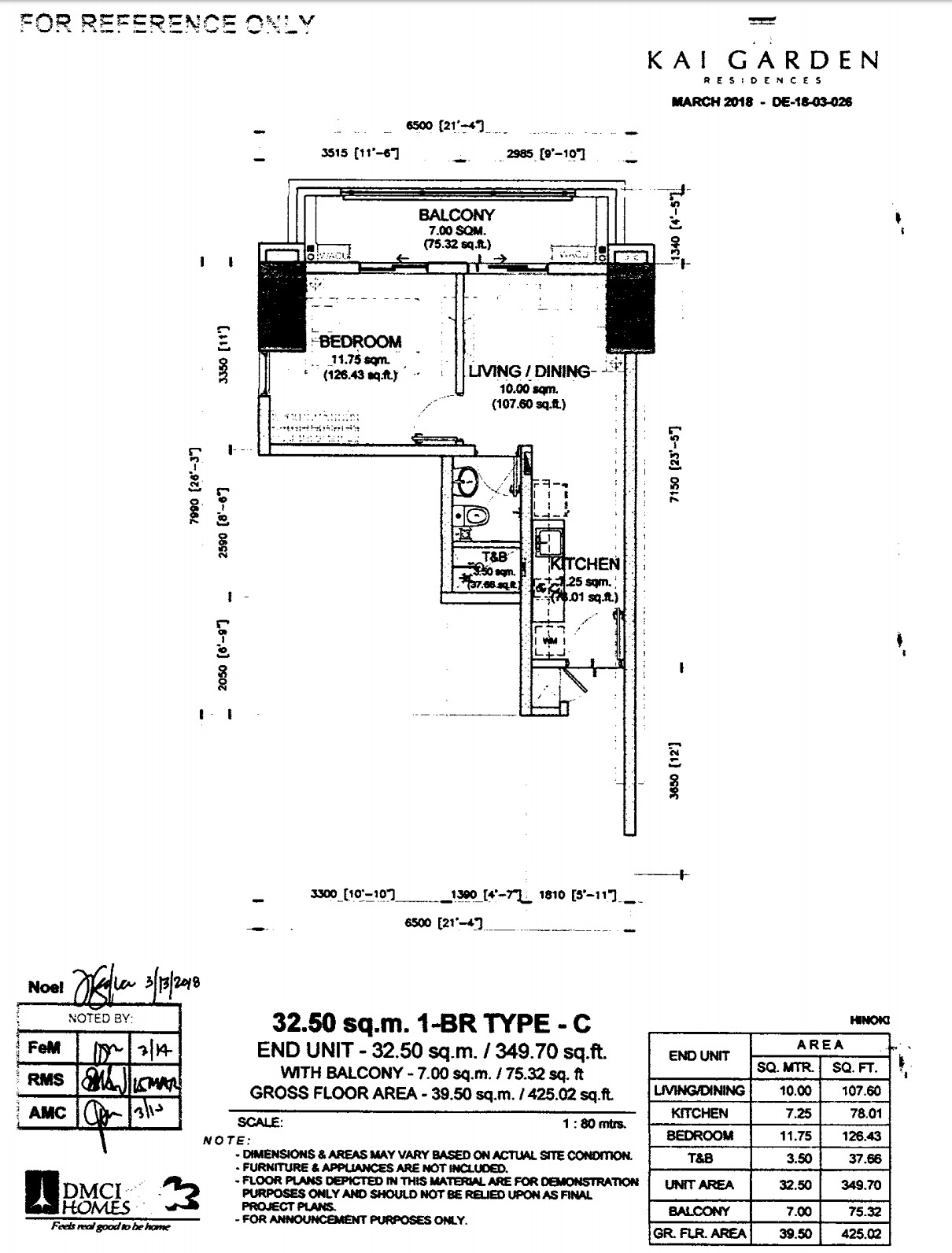Caption: 

This detailed, yet challenging to decipher image appears to be a printed floor plan of "Kai Garden." Presented entirely in black and white, the small and somewhat faded print displays a layout for a "One Bedroom Type C End Unit with Balcony," measured at 39.5 square meters (425 square feet) of gross floor area, totaling 700 square meters. At the top, the note "for reference only" is visible, emphasizing the illustrative nature of the diagram. The floor plan reveals a cohesive design where both the bedroom and living room open onto a shared balcony, offering a seamless indoor-outdoor transition. A compact bathroom and a kitchen area are also illustrated, beside what seems to be a modest storage space. The layout annotations include labels for living, dining, kitchen, bedroom, toilet and bath (T and B), unit area, and balcony, completing the architectural outline of this end unit.